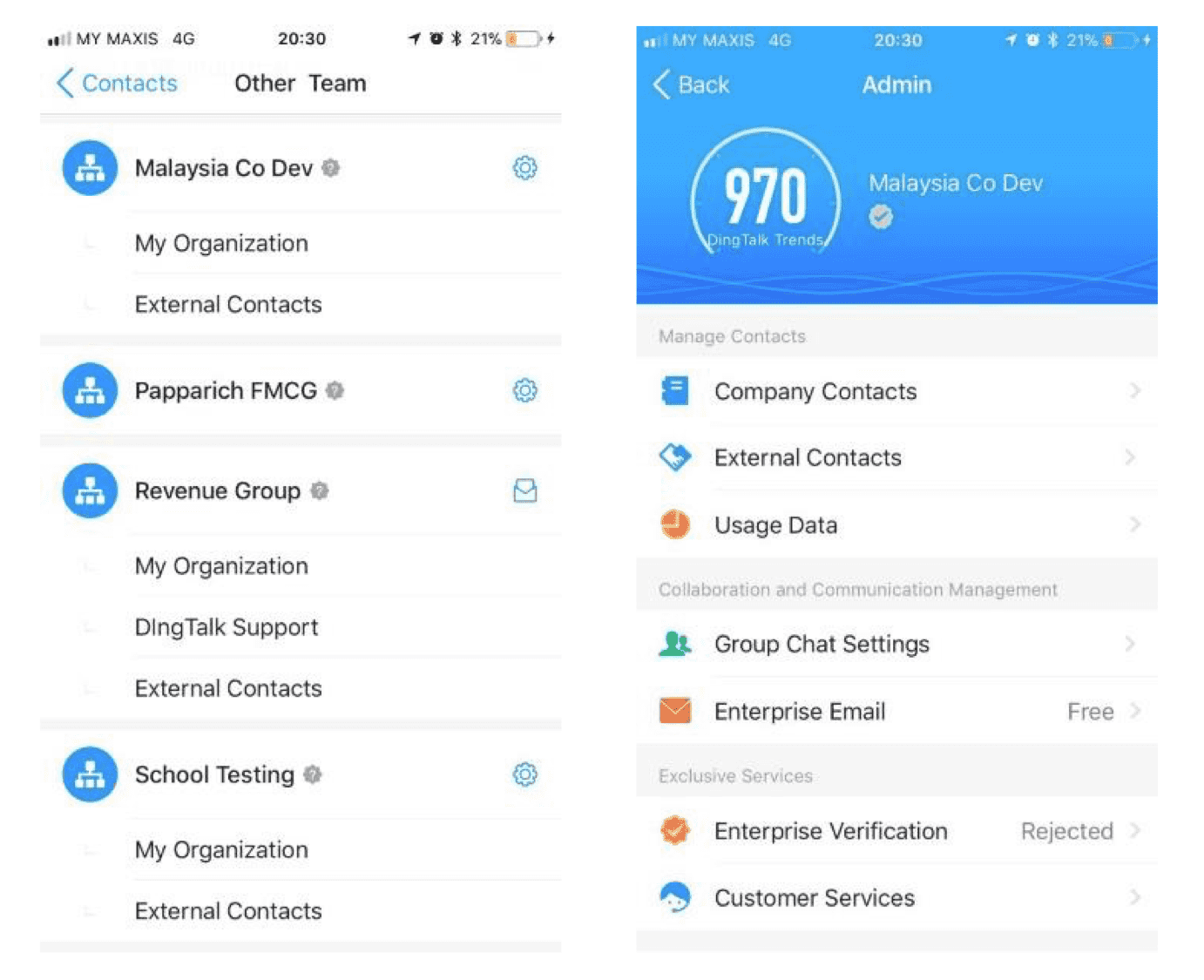The image displays two side-by-side screenshots from a phone, illustrating distinct yet related functions of a business organizational tool.

On the left side, there is a contact book featuring four different contacts, each with sub-contacts organized underneath the main entries. The main titles include categories such as "My Organization," "External Contacts," and specific groups like "Paparich," "FMCG," "Revenue Group," "DigTalk Support," and "School Testing."

The right side shows the main page of an administrative app. At the top, it reads "Admin," followed by a score, "970." Adjacent to the score is a label that says "Malaysia Code D.E.V.," suggesting company development or related information. Below this are various headers and categories for managing business operations. The "Manage Contacts" section includes "Company Contacts," "External Contacts," and "Usage Data." Further sections are titled "Collaboration and Communication Management" (covering "Group Chat Settings" and "Enterprise Email") and "Executive Services" (listing "Enterprise Verification" and "Customer Services").

Together, these screenshots depict a comprehensive view of a business management app designed to streamline contact organization and communication within a company.